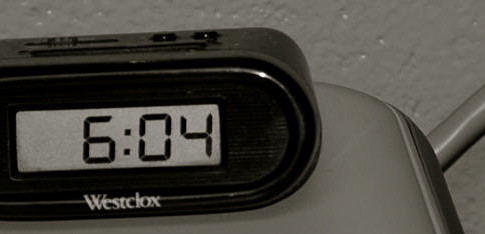This is a detailed photo of a somewhat retro digital alarm clock. The clock is branded "Westclox," spelled W-E-S-T-C-L-O-X in white letters, prominently displayed on the lower part of its clear front. The clock itself is black with an oblong or oval shape, and it features a small silver ring that outlines its display. The digital screen shows the time as 6:04 in black numbers on a gray background. 

On top of the clock, there are two small black buttons, and a lever to the left that can presumably be slid left or right, possibly for setting an alarm or other functions. An additional feature is a short antenna sticking out, suggesting it may have radio capabilities.

The clock rests on the cushion of a gray chair, described by different observers as possibly being patent leather or part of a straight-back dining room chair. Behind the clock is a white textured wall with small indented circles, adding depth to the background. The setting creates a mix of functional design and homey background details, highlighting both the clock's utilitarian and nostalgic aspects.